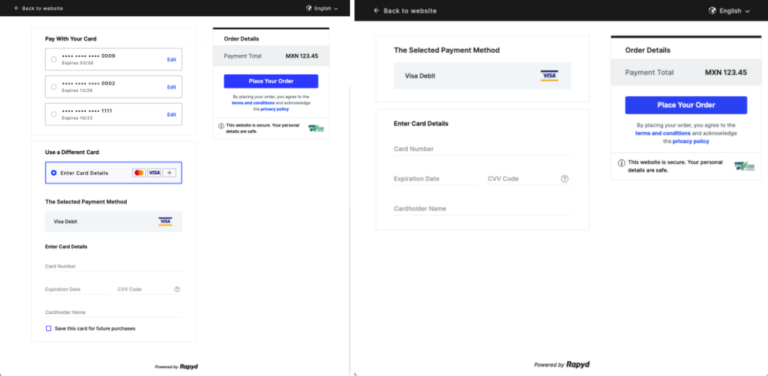Here is the cleaned-up and detailed caption for the image:

---

**Screenshot Depictions of a Website Checkout Process**

This image features two side-by-side screenshots detailing the checkout process on a website. Both screenshots are somewhat pixelated, rendering much of the text illegible. Below is a more focused description of each segment:

**Left Screenshot:**
- **Credit Card Options:** This section lists three credit card choices, with placeholder numbers that do not represent real cards. The cards are labeled generically.
- **Card Entry Box:** Below the card options is a selection box outlined in blue, indicating the choice to either use a listed card or enter new card details. The entry fields include:
  - Card Number
  - Expiration Date
  - CVV
  - Cardholder Name
  - An option to save the card for future purchases
- **Selected Payment Method:** The default payment method displayed is Visa Debit, shown in a gray box.
- **Footer Tag:** There is a footer tag, though it is not legible.

**Right Screenshot:**
- **Consistent Selection Options:** Similar to the left screenshot, it displays the Visa Debit as the selected payment method, also within a gray box, along with fields to enter card details.
- **Order Details Section:** This includes a breakdown of the payment totaling in Mexican Pesos (MXN), specifically listed as "1, 2, 3, 4, 5." The “Place Your Order” button is emphasized in blue with white text.
- **Footer Texts:** More legible compared to the left screenshot, stating:
  - "Powered by ROPYD" in the footer.
  - A disclaimer mentioning that by placing the order, the user agrees to the terms and conditions, and acknowledges the privacy policy.
  - Assurance that the website is secure, indicating that personal details are safe.
- **Logo and Additional Text:** There is a logo composed of different shades of green, but its specifics are not clear.

---

This caption aims to describe the visual elements and functionalities depicted in the screenshots comprehensively.